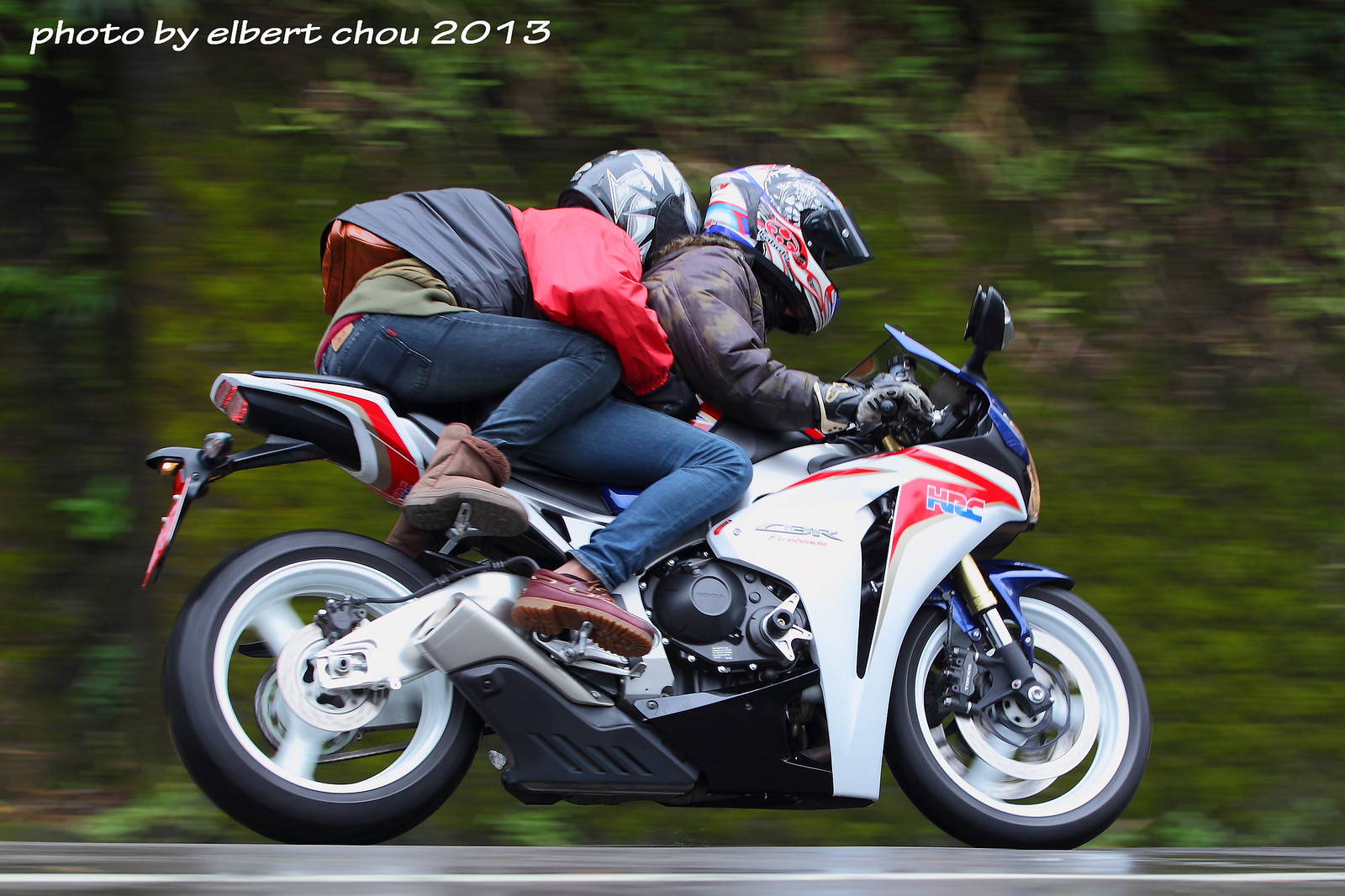The image captures a dynamic moment of two people speeding on a white motorcycle with red and blue trim. The motorcycle's rims are white, matching its overall sleek aesthetic. Both riders are leaning forward, enhancing the sense of speed, which renders the background of green trees and foliage into a blurred mix of greens. The dark gray pavement is marked with a white stripe, adding to the sense of motion.

The rider in front is dressed in a brown leather jacket, blue jeans, and brown shoes. The rider behind, dressed in a red jacket over a green shirt, also wears blue jeans and brown shoes. Both riders sport helmets with colorful graphics; the front rider's helmet includes blue, white, and red elements. The rear rider holds on tightly with their right arm wrapped around the front rider and carries a small backpack.

In the top left corner, the image is credited with the text "Photo by Albert Chow, 2013," adding a timestamp and author signature to this thrilling moment frozen in time.